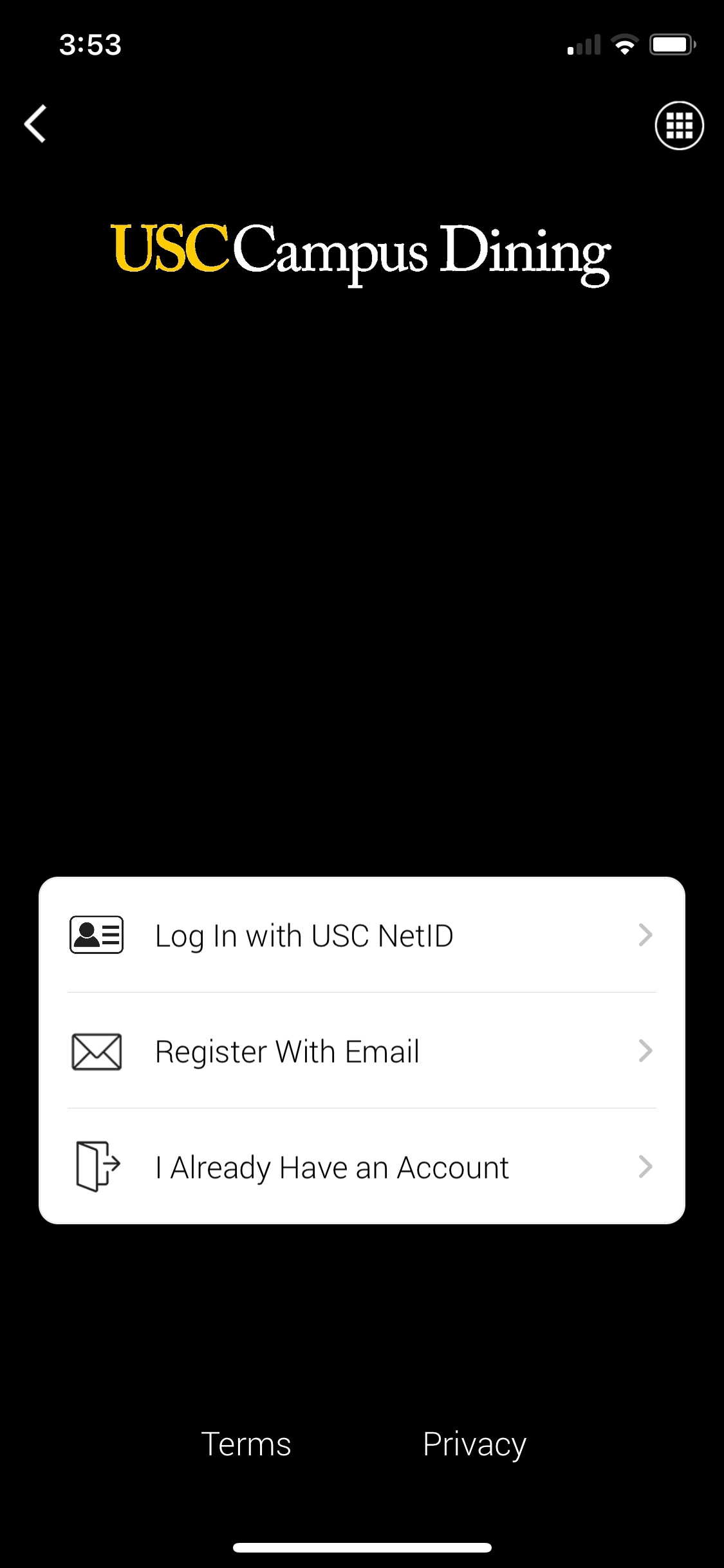This image is a screenshot of a smartphone menu interface that predominantly features a black background with white text. At the top of the screen, the current time is displayed in the upper-left corner as 3:53, though there is no indication of whether this is AM or PM. Adjacent to the time, a data information indicator is present. Below this, on the left side, a white, left-justified arrow suggests the option to navigate back within the application. Centered beside the arrow, there is an iconic menu item represented by a circle containing several tiny squares, indicating that additional menu options can be revealed by clicking on it.

The main heading on the screen reads "USC Campus Dining," with "USC" in yellow text and "Campus Dining" in white, though it appears as a single continuous word. Below this title, a large empty black space dominates the center of the screenshot.

Further down, a subtext menu appears, consisting of three rows of thin black text on a white background, each accompanied by iconic representations in the left-hand column. The menu options are as follows:

1. "Log in with USCnetID"
2. "Register with email"
3. "I already have an account"

At the very bottom of the screen, in white text against a black background, the options "Terms" and "Privacy" are listed.